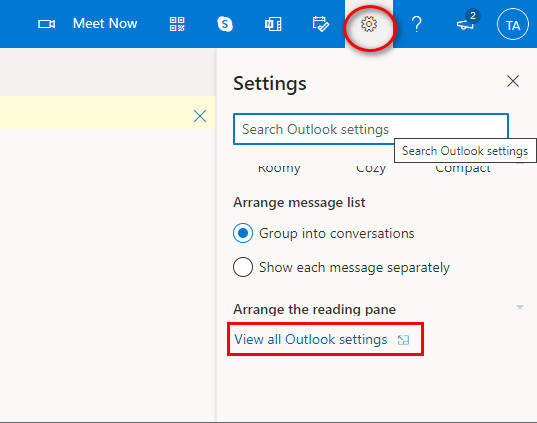The top of the image features a camera icon alongside the text "Meet Now," accompanied by several square icons. Among these icons are the recognizable Skype symbol, a large "N," a movie or picture-like square, a calendar icon with a check mark, a white square, and a gear icon in the center. Encircling the edges is a red circle. Additionally, there is a blue square containing a question mark, a megaphone icon, and a blue circle with the number "2" at its center. A white circle labeled "TA" is also present, along with a rectangle on the left that contains rows aligned to an "X" shape. Other visible elements include settings options and a blue "N" with the prompt "Search Outlook settings."

The screen further includes words like "roomy," "cozy," "compact," "breakfast," "arrange," and "message list." A blue circle labeled "Group and conversations," the text "circle and size is nothing," and the option "Show each message separately" are indicated. The layout also features directions to "Arrange the reading pane." The view is bordered in red with an area at the bottom displaying the text "View all Outlook settings" in blue. A divider line or border is drawn at the bottom of the screen to provide further separation within the interface.